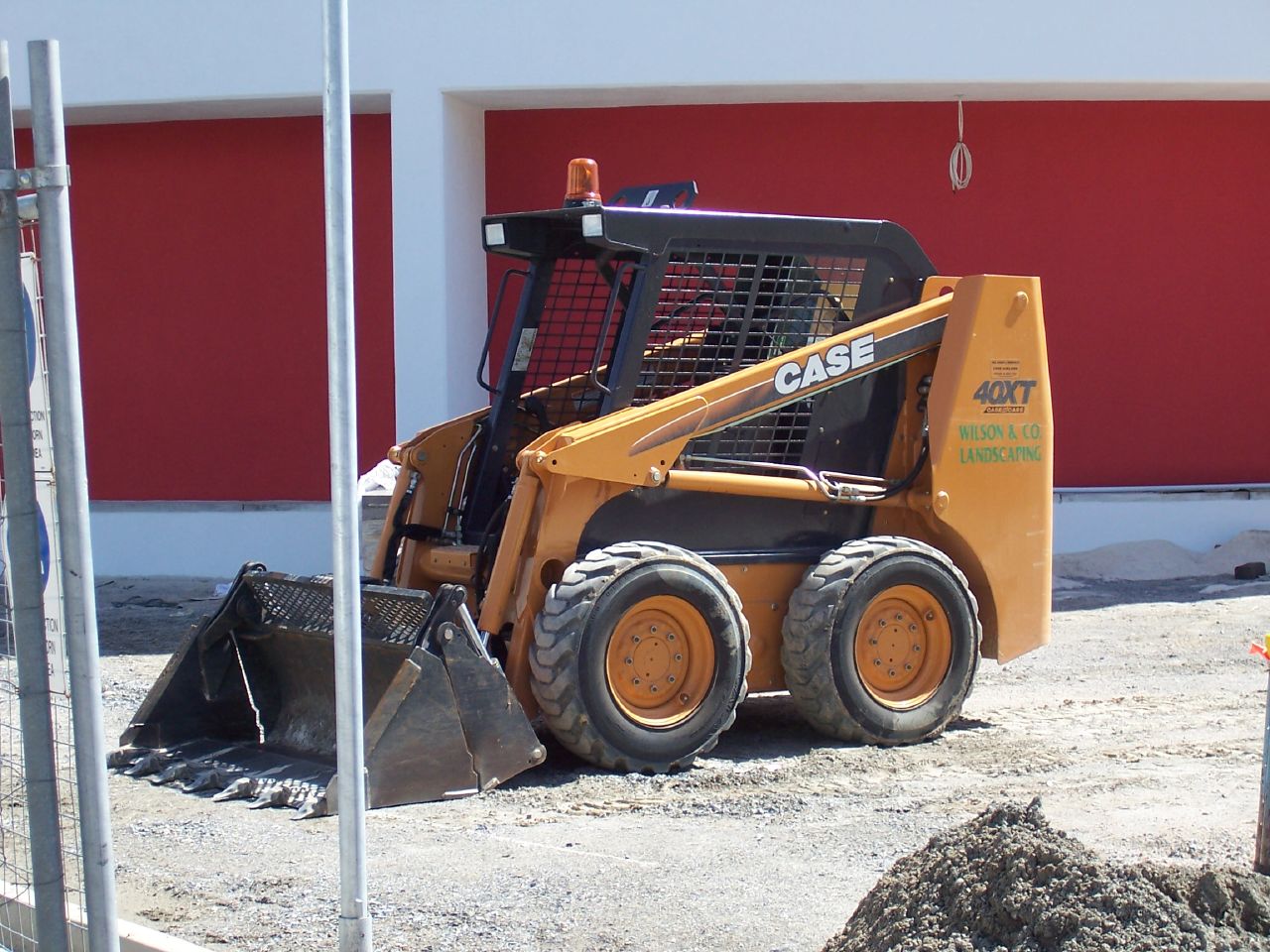This photograph, taken at a brightly sunlit construction site, captures a yellow bulldozer resting motionless on a ground covered in gray soil or gravel. The bulldozer, with its distinctive construction yellow paint, features a front scooper, two large black wheels visible on the side, and a black cage where the driver operates. The side prominently displays the text "CASE" in white letters, along with additional identifiers such as "KS40XT" and "Wilson & Co Landscaping." To the left of the bulldozer, a gray chain-link fence and a metallic pole are visible. In the background stands a red and white building characterized by horizontal and vertical beams, contributing to the scene's industrial atmosphere. The photograph, captured in bright morning or midday light, also includes a nearby pile of dirt, indicating that work may not yet have commenced for the day.